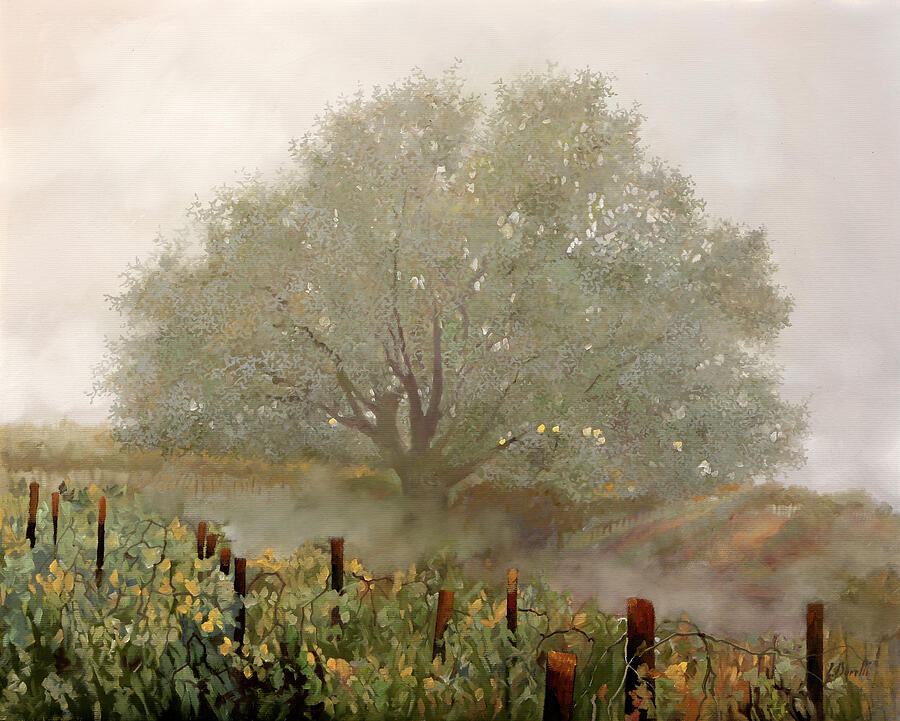This vibrant color painting captures an expansive scene centered around a colossal tree that dominates a vast field. This tree, possibly a walnut tree, stands majestic and towering over its surroundings with an intricate network of extensive branches covered in greenish-gray foliage, accented with touches of yellow fruit. The imposing tree fills up approximately 75 percent of the composition, drawing the viewer's eye to its grand stature against the hazy, fog-swept sky typical of the California Central Valley.

In the foreground, partially obscured by the low-lying fog, a weathered fence constructed of rusted metal posts and wire, possibly barbed or for supporting grapevines, runs through the scene. These posts are enveloped by tall grass and vines, hinting at the passage of time and the slow encroachment of nature. The landscape also features rows of plowed earth or dirt pathways weaving behind the tree, suggestive of agricultural activity. The distant hills and gently rolling fields, dotted with what may be a faint outline of a house, further enrich the bucolic atmosphere of this painting, evoking a sense of timeless rural tranquility in the misty air.